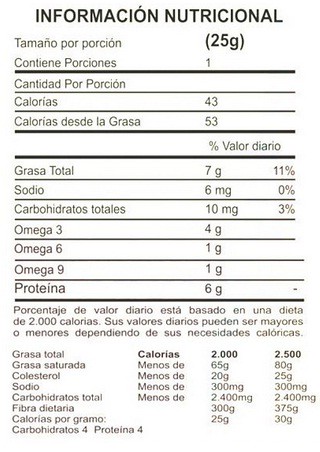This is an image of a nutritional label written in French. The label bears the heading "Informations Nutritionnelles," indicating nutritional information. Although the text is primarily in French, certain universal nutrient names are decipherable, such as "Oméga-3," "Oméga-6," "Oméga-9," and "Protéine" (Protein), signifying the presence of these nutrients. Below the main nutritional facts, there is a paragraph in French that elaborates on the nutritional elements and ingredients contained within the product. The product's weight is specified as 25 grams. The front of the packaging is not visible in the image provided.